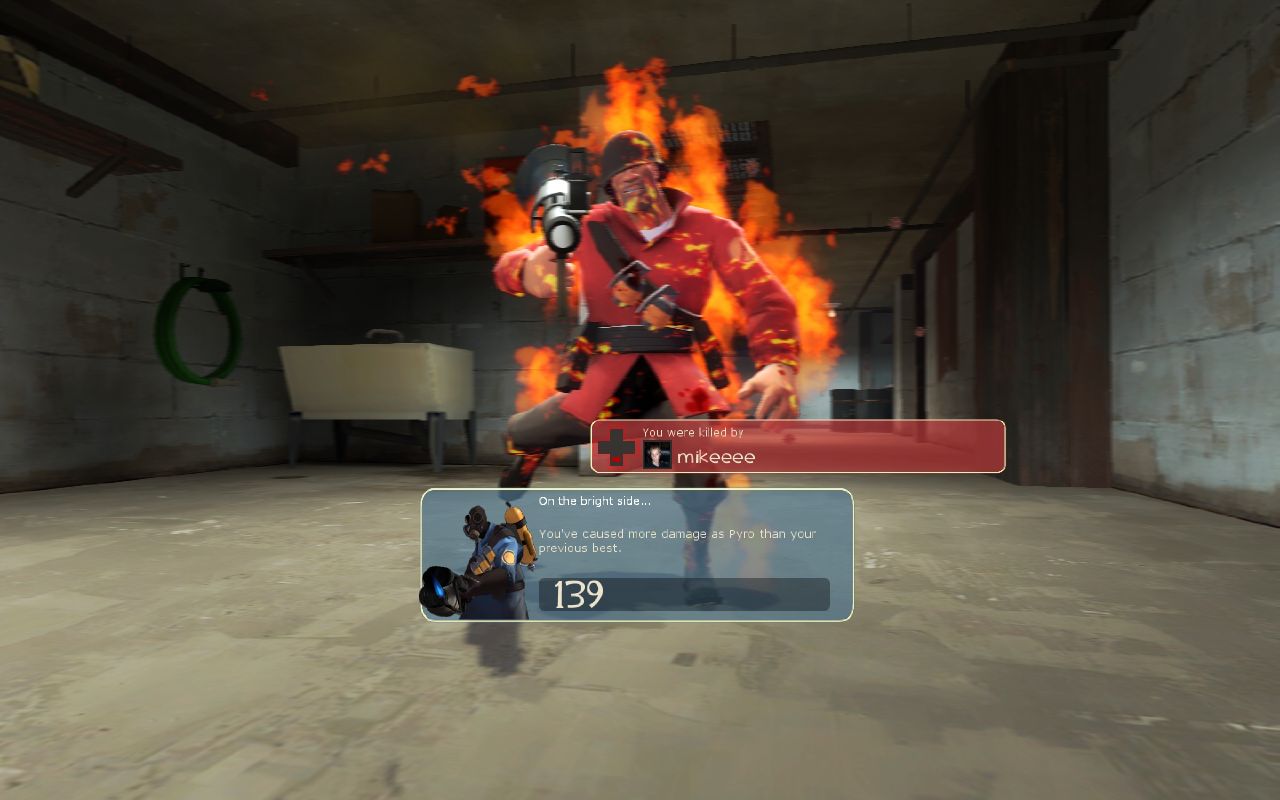This detailed screenshot from the video game Team Fortress 2 captures a dramatic moment featuring the character Soldier, who is engulfed in flames. Soldier, recognizable by his red coat, gray pants, and helmet that obscures his eyes, is prominently positioned in the center, standing on one foot while the other leg juts out awkwardly. He wields a large weapon, likely a rocket launcher, pointed directly at the viewer. The scene implies intense action as flames erupt from his body, indicating that he is on fire.

In the foreground, text overlays convey crucial information: "You were killed by Mike E." and "On the bright side, you've caused more damage as Pyro than your previous best, 139." These messages not only indicate the cause of Soldier's demise but also highlight a personal achievement in gameplay.

The background depicts a sparse, warehouse-like environment with cement floors and metal beams. Notable elements include a white tub or sink in the left corner, a green hose hanging nearby, and a rope on the wall. The room appears dimly lit, contributing to the gritty atmosphere of the scene. The layout is emphasized by the landscape orientation of the screenshot, which enhances the immersive experience of this intense moment in Team Fortress 2.